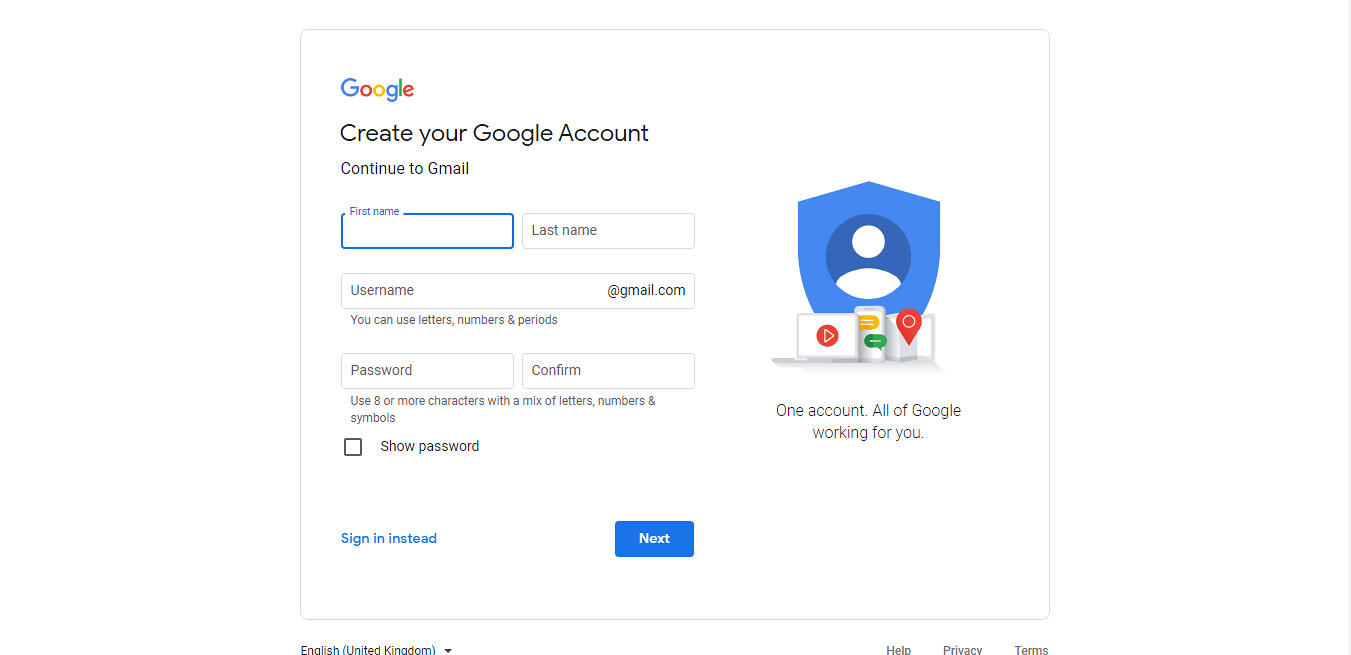This image is a detailed screenshot of a Google account creation page. The page is square-shaped, and prominently features Google's logo—a shield—on the right-hand side, accompanied by icons of a tablet, computer, and mobile phone in the center. Below these icons, a slogan reads: "One account. All of Google working for you."

In the upper left corner, the colorful Google letters catch the eye, followed by a headline that says, "Create your Google Account." Below this, there is an option labeled "Continue to Gmail." 

The form begins with spaces to input your first and last name. Following these fields, users are prompted to choose a username, accompanied by a note indicating that letters, numbers, and periods are allowed. Below the username field are two rectangular blocks for the password: the first for entering and the second for confirming it. Instructions for the password are provided, specifying to use eight or more characters with a mix of letters, numbers, and symbols. 

An option to show the password is available via a small square block. Below all this in black letters is the link "Sign in instead" for those who already have an account. To the right, there is a prominent rectangular blue box with white text that reads "Next."

Finally, at the bottom of the image, various clickable options are available including "English (United Kingdom)," "Help," "Privacy," and "Terms."